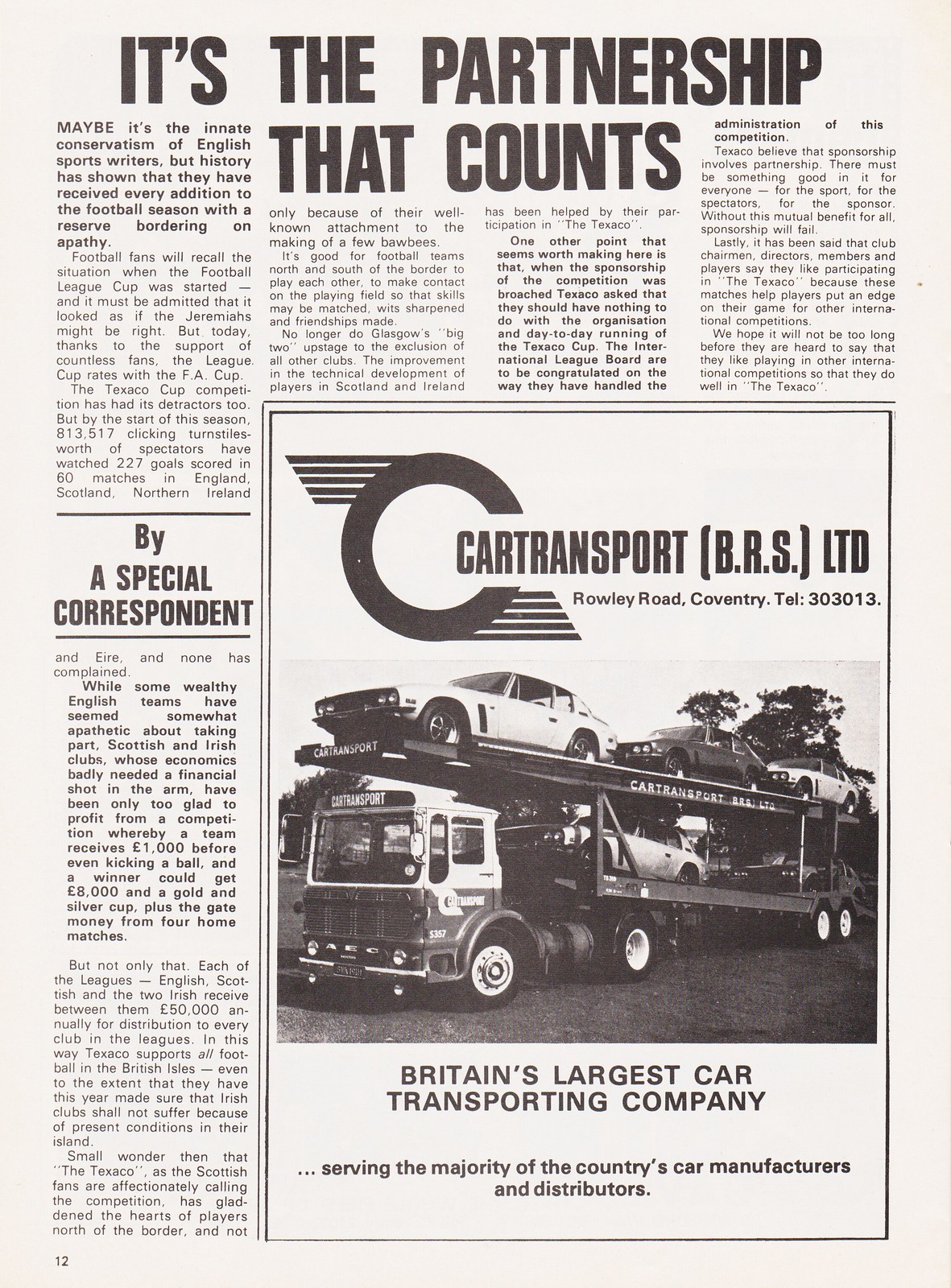The image is a scanned copy of a football program or magazine page with a white background and multiple lines of black text. The article, titled "It's the Partnership that Counts" by a special correspondent, discusses the historically conservative reception of new additions to the football season by English sports writers. It highlights the initial apathy towards the Football League Cup, which eventually gained popularity among fans, leading to a significant spectator turnout and numerous goals scored. Adjacent to the article, there is a large advertisement spanning three columns featuring Car Transport BRS Ltd., Britain's largest car transporting company. The ad includes an image of a tow truck carrying multiple cars and details the company's service to the majority of the country's car manufacturers and distributors. Also, prominently displayed is the company’s address at Crowley Road, Coventry, along with a contact telephone number.